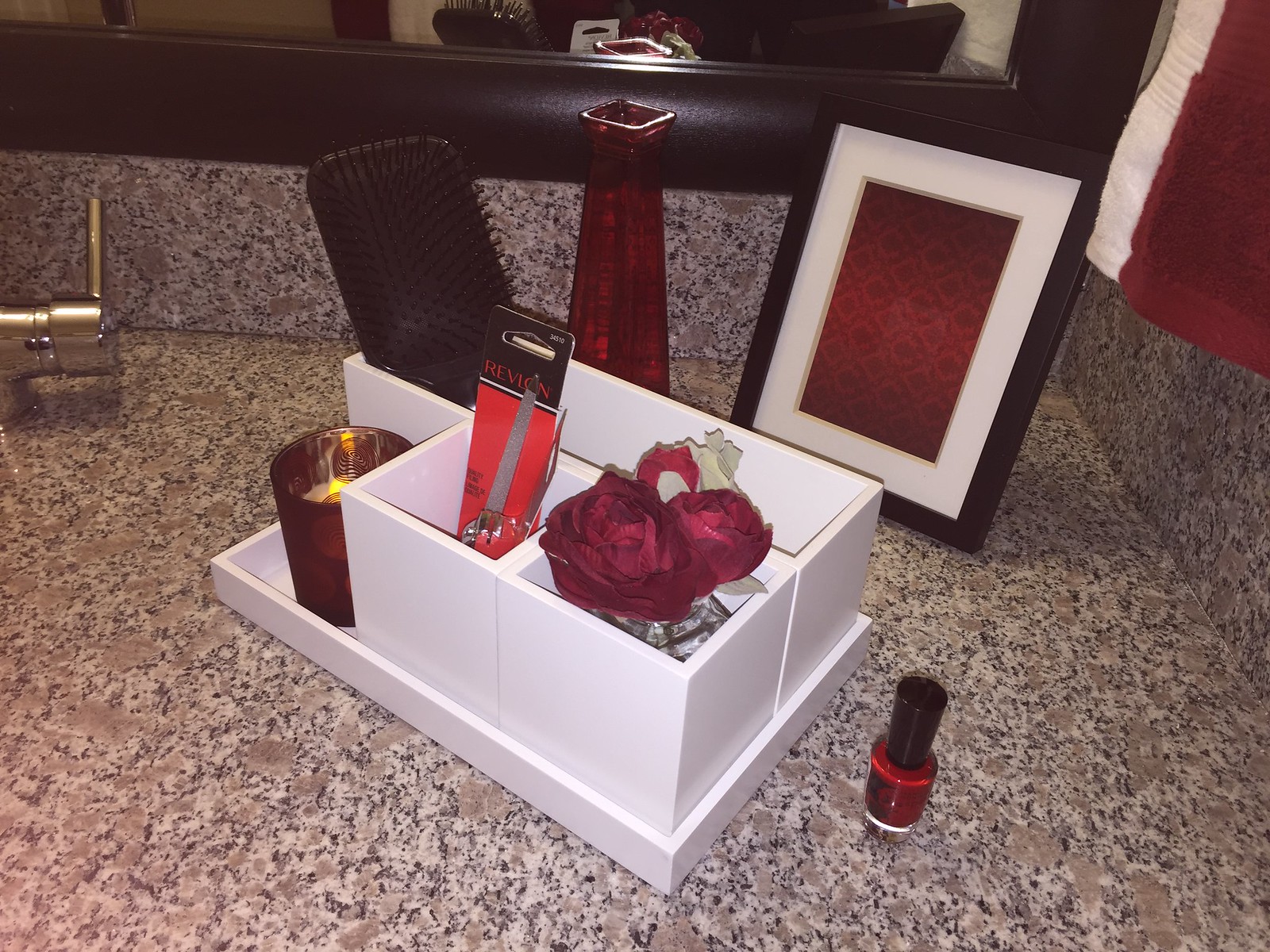The photograph captures a detailed view of a bathroom countertop made of speckled grey and black granite. On the left side, the chrome faucet sits adjacent to an unseen basin. Directly above the countertop, the bottom edge of a thick, chocolate-brown wooden mirror frame is visible, spanning the width of the counter, and reflecting the elegant bathroom decor.

On the right, two towels—a white one and a maroon-red one—hang neatly. The countertop itself features a variety of items. Prominent among them is a sturdy, wooden display box with multiple compartments. The box's leftmost compartment is open, revealing a maroon-colored glass container with a lit candle inside. 

Behind the wooden box, there is a wide, square-shaped black hairbrush with plastic bristles, emphasizing everyday functionality. A maroon-colored glass vase, devoid of flowers, stands near the back, adding a pop of color and elegance.

To the right of the vase, a vertically-oriented rectangular picture frame with a dark chocolate-brown outer frame and a white inner frame stands. Instead of a photo, the frame displays maroon-red patterned paper, enhancing the room's sophisticated color scheme.

Returning to the wooden box, inside one of its compartments, a Revlon nail care kit is visible, complete with a nail file and a cuticle pusher, packaged in characteristic black and red Revlon branding. On the far right, two delicate, maroon-red fabric roses lie beside a maroon-red nail polish bottle with a long black cap, contributing to the overall aesthetic coherence and hinting at the luxurious attention to detail within the space.